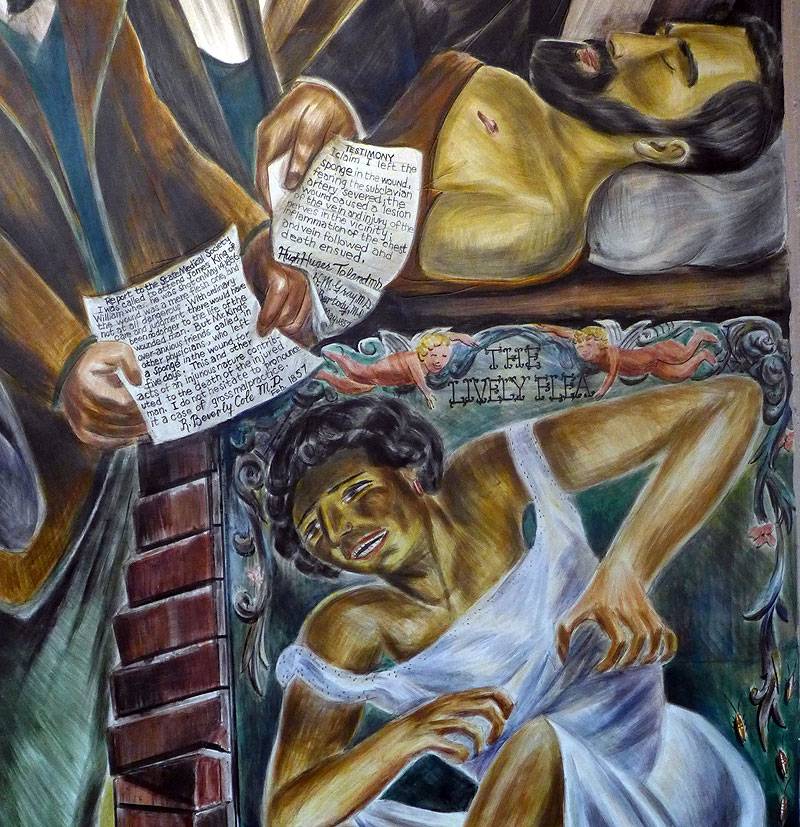The image is a square oil painting, stylistically realistic with a touch of cartoon-like qualities, bordered with bricks on the left-hand side. At the top right, a gold-skinned man with long black hair and a black goatee lies on a wooden slab, his head resting on a soft, light gray pillow. He appears to be asleep or possibly dead, his eyes closed and a mysterious stamp mark on his chest. Above him, a black-suited arm extends, holding a note that reads "testimony," with partial text claiming "I left this sponge in the wound."

On the upper left of the painting, there's a cropped figure wearing a brown jacket, also holding a piece of paper inscribed with indistinct English text. Below this somber scene, in the lower right-hand corner, a black woman, depicted in great agony, is seated with her right arm holding something under her white dress. She has black hair and crossed legs, and the text "The Lively Flea" is written above her. The painting exudes a narrative quality, blending elements of medical and emotional turmoil.